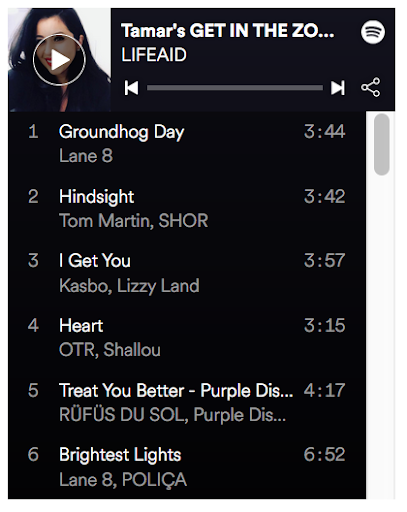**Detailed Caption:**

This is a detailed screenshot of a Spotify playlist featuring a variety of songs from different artists. The playlist prominently includes a track by the band LifeAid titled "Tamar's Get In The Zoo." To the left of the song title, a small video insert from the corresponding music video is visible, while the Spotify logo is displayed to the right, signifying the platform. Directly below the band and song title, there is a search bar where users can search for more music.

The playlist includes six distinct songs listed below the search bar:
1. "Groundhog Day" by Lane 8, which has a duration of 3 minutes and 44 seconds.
2. "Hindsight" by Tom Martin and Shore, lasting 3 minutes and 42 seconds.
3. "I Get You" by Kazbo and Lizzy Land, with a length of 3 minutes and 57 seconds.
4. "Heart" by O.R.T. and Shalhoub, running for 3 minutes and 15 seconds.
5. "Treat You Better" by RÜFÜS DU SOL and Purple Disco Machine, extending for 4 minutes and 17 seconds.
6. "Brightest Lights" by Lane 8 and POLIÇA, which is the longest track at 6 minutes and 52 seconds.

On the right side of the playlist, a scroll bar is also visible, allowing users to navigate through additional songs. The interface features a sleek black background with white text for a modern and clear visual contrast.